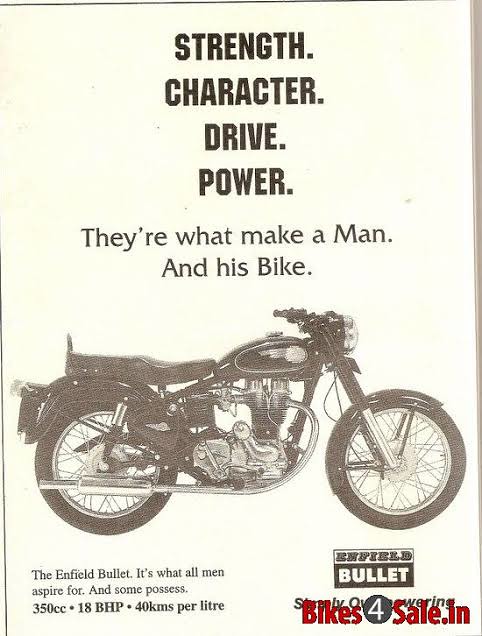The image appears to be a dated advertisement or magazine page with an off-white, worn background. At the top center, bold black letters spell out "Strength, Character, Drive, Power" in a vertical arrangement. Below this, the text reads, "They're what make a man and his bike." The centerpiece of the image is a black and white side-view photograph of a motorcycle, specifically an Enfield Bullet. Detailed specifications are listed below the image: "350cc, 18 bhp, 40 km per liter." In the bottom right corner, red text advertises "bikesforsale.in." The overall feel of the image is nostalgic, evoking a sense of rugged masculinity and timeless aspiration.